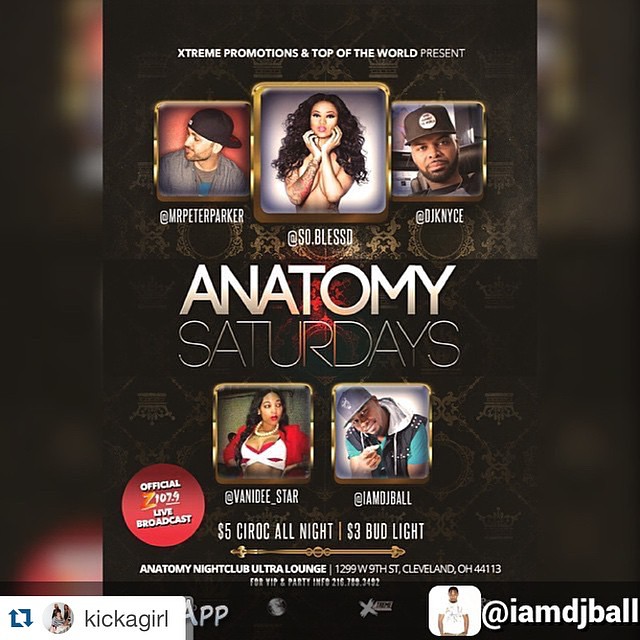This social media post is an advertisement for an event named "Anatomy Saturdays," presented by Extreme Promotions and Top-of-the-World. The background is black, featuring images of five African-American actors, each accompanied by their hashtags. The top row includes Mr. Peter Parker, who is wearing a backward hat; So.Blessed, a woman with long black hair, partially nude but covering her breasts with her arms and hands around her cheeks; and DJ Kents, a black man also wearing a hat. Below them are Vanity Star, a black woman in a halter top, and IM J Ball, another black man with a hat. There is a red circle indicating an "Official Live Broadcast" by Z107.9. The event offers $5 Ciroc and $3 Bud Light all night, and it's hosted at the Anatomy Nightclub Ultra Lounge in Cleveland, Ohio. The post is tagged with #IAmDJDJBall and has been reposted from @kickagirl.